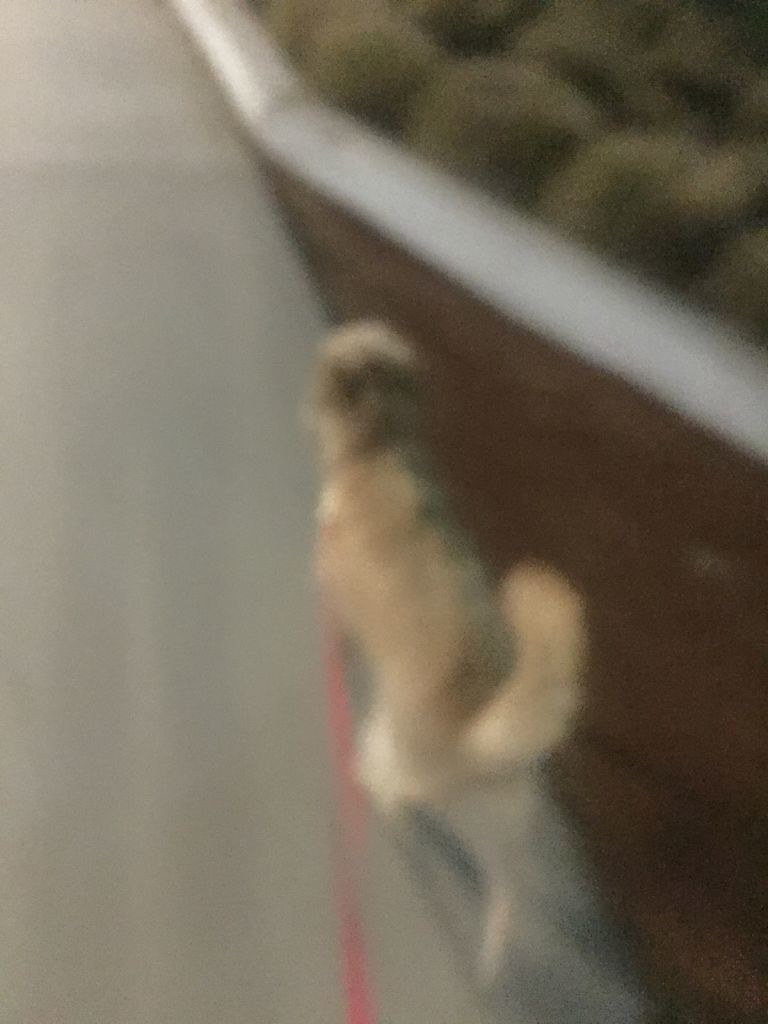In this out-of-focus photograph, a tan-colored animal is captured in mid-climb at the edge of a vertical surface, reminiscent of a fence or a rock formation commonly seen in a zoo. Though the entire image is heavily blurred, the outline of the animal's body suggests a long, feline form. The creature's right hind leg is extended downward, while its left hind leg remains obscured beneath its body. A distinctive plume-like tail arches upward, reminiscent of a squirrel's but indicating a different animal. The blur renders fine details indistinguishable, but the overall posture and form of the animal suggest an active moment frozen in time.